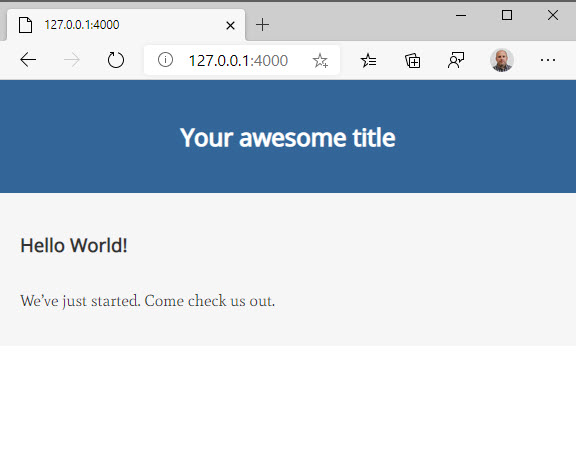A detailed screen capture of a web browser displaying a local development environment for a nascent website. The single open tab shows the URL "127.0.0.1:4000," indicating that the user is accessing a local server for development purposes. Navigation controls include an active back arrow, a grayed-out forward arrow, and a reload button. To the right, an "i" within a circle provides information related to the local server address. The user profile icon is visible in the UI. The browser's prominent blue header bar features the placeholder text "Your Awesome Title." Below, the main content area greets visitors with "Hello, World!" followed by the message, "We've just started, come check us out." This setup suggests that the user is either testing the initial stages of a website or exploring a template design.